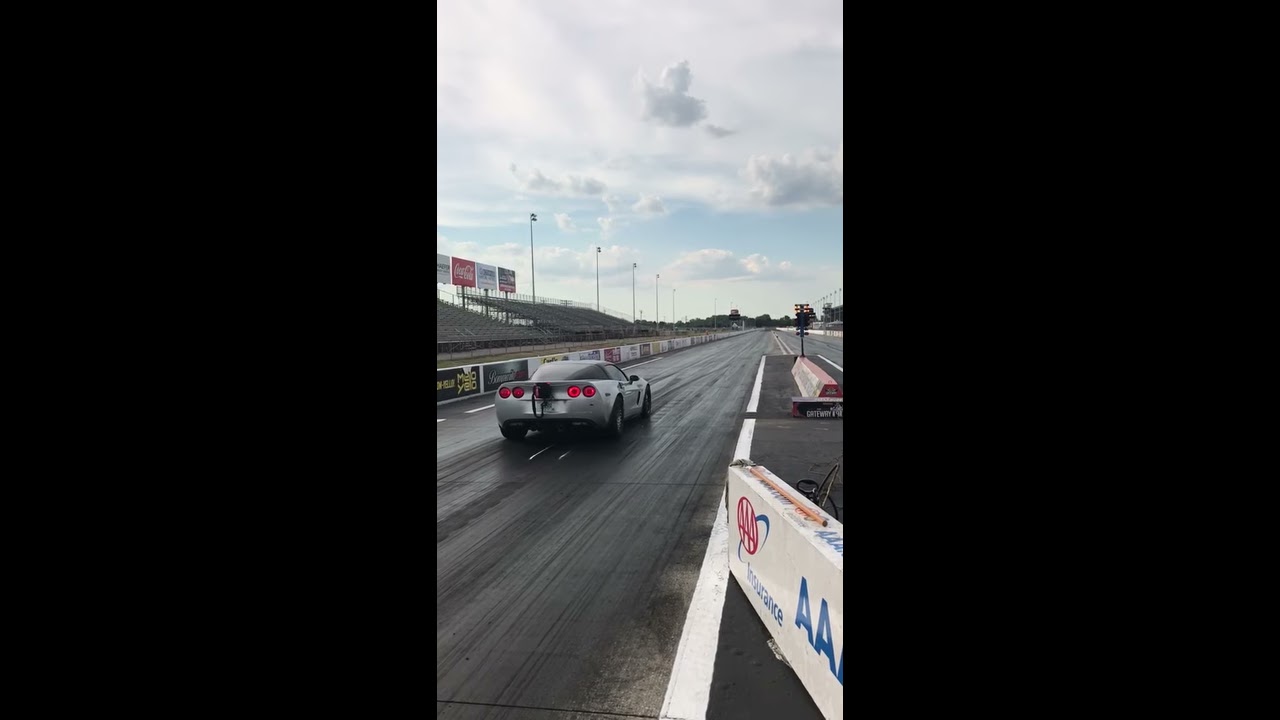The image captures a daytime scene at a drag racetrack with the focus on the straight strip of the track. On the left lane, a silver and gray two-door sports car with four rear red lights is positioned, facing away from the camera. This car is the only one on the track. The track appears wet and reflective, with solid white lines denoting the edges of each lane. The left side of the racetrack features several empty bleachers with various advertising signs, the most noticeable being a red Coca-Cola sign in the center. The right side of the image shows a barricade adorned with a AAA Insurance logo. The sky is a light blue, scattered with white clouds, enhancing the sunny yet tranquil atmosphere of the scene.